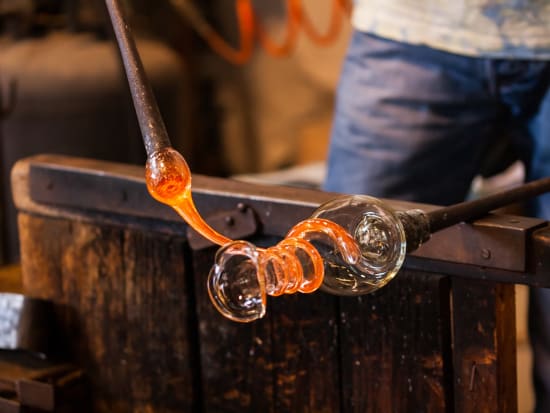The image depicts a scene of glassmaking in progress. A man, whose lower half is visible, stands in a workshop wearing blue jeans and a white shirt. He is engaged in the intricate process of creating a coiled glass figure. His work area features a metal top resting on a wooden base. Using two rods, he manipulates softened orange glass, tempered and malleable from the heat, on the end of one rod. The orange glass is being wound around a white glass structure that resembles a vase. The man’s left hand stabilizes the vase with a rod, while his right hand skillfully wraps the heated glass around it, forming a spiral pattern. The space around him is filled with the warm glow of the glassmaking process, emphasizing the concentration and craftsmanship required in this precise art form.